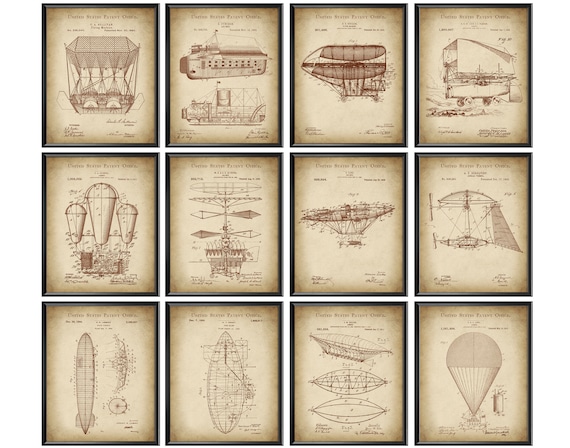The image is a detailed photograph of 12 rectangular pencil sketches, all enclosed in black frames and arranged in a grid with three rows and four columns. The sketches, rendered on aged, brownish-beige paper, illustrate various imaginative designs of early flying machines, ranging from zeppelins and hot air balloons to rudimentary airplanes. Each image showcases unique and sometimes fantastical aeronautical concepts, such as a plane with a propeller unusually positioned several feet above its body in a manner resembling an intake port, and an oblong, submarine-shaped machine with metal exterior and individual windows. There is also a design of a zeppelin's passenger section and another of a boat-like flying contraption with a tent structure. Text is visible on each sketch but is too small and poorly contrasted to read easily, suggesting these might have been conceptual patent submissions. The intricate details and variety of designs highlight the artist's creative envisioning of early aviation technologies.